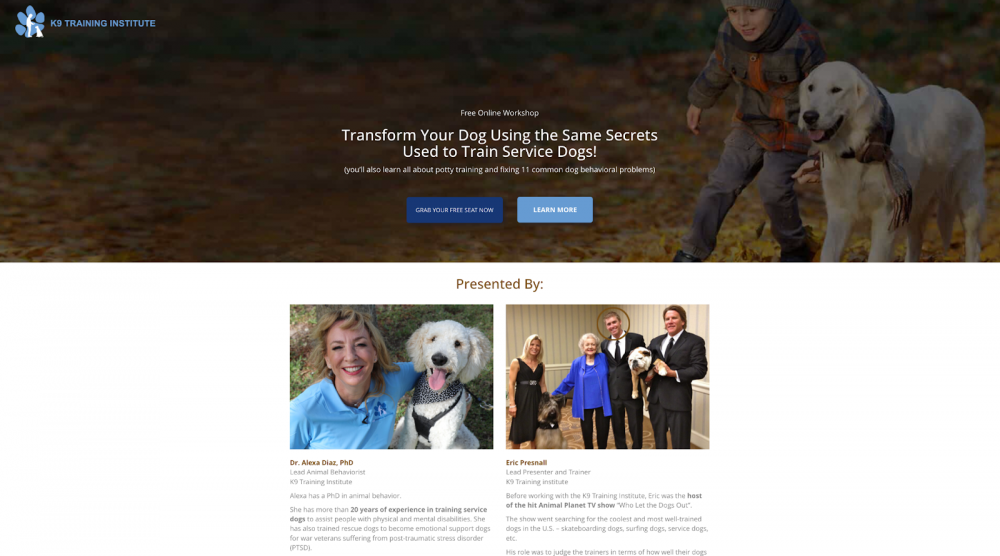In this screenshot, there is a promotional banner for a program titled "Transform Your Dog Using the Same Secrets Used to Train Service Dogs." The main image features a little boy with his Labrador, smiling and showing a playful bond. Below this, there are two smaller pictures. The first smaller image showcases a woman, wearing a light blue shirt and holding a poodle-like dog. Her warm smile, combined with her professional demeanor, suggests she might be a doctor specializing in veterinary care. The second smaller image features two gentlemen in black suits standing on either side of actress Betty White, who is surrounded by two dogs. A woman in a sleeveless black dress stands beside them. A circle highlights the head of one of the men, who has his arm affectionately wrapped around Betty White.